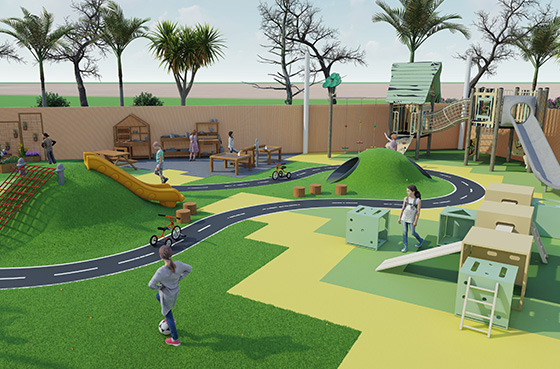In this highly detailed computer-generated rendering of a playground, a vibrant and meticulously designed park area is depicted. The ground is primarily covered with a green turf, punctuated by patches of yellow and light green hard surfaces. A meandering gray road with white lines cuts through the playground, curving around a small grassy hill. Various play structures populate the area, including a yellow slide descending from one of the hills, a red climbing net, monkey bars, and several little houses for imaginative play.

Children can be seen joyfully interacting with the equipment, while a few adults, presumably parents, supervise in the background. The backdrop features a mix of lush greenery transitioning into a peachy-tan hue, populated by an assortment of trees, including palm trees, and lower bushes, all enclosed by a wooden fence. Overall, this well-developed and inviting park, likely the brainchild of a landscape architecture firm, provides a detailed and enticing vision of an ideal recreational space for children.